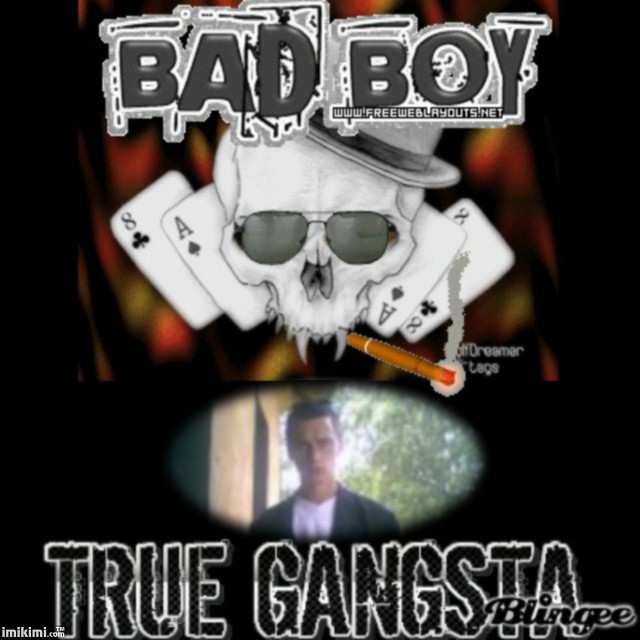The image appears to be either the cover of an album or a promotional flyer, predominantly showcasing dark hues with a gradient that becomes lighter towards the center. Splashes of red, orange, and yellow add vivid contrast to the background. Prominently displayed at the top is the bold phrase "Bad Boy" in striking black letters. Central to the composition is a grayscale drawing of a human skull, accentuated with black sunglasses and a gray top hat. The skull's teeth are notably sharp and menacing, akin to a vampire's fangs. It is smoking a cigar that blends characteristics of both a cigarette and a cigar. Flanking the skull are playing cards: the Eight of Clubs and the Ace of Spades are positioned behind it, each repeating on either side. Below the skull is an oval-shaped photograph depicting a serious-looking young white male with short brown hair, clad in a white shirt and a dark jacket, set against a backdrop of trees. The image is completed with the inscription "True Gangsta" beneath the photograph. The flyer also features a web address, www.freeweblayouts.net, indicating its digital origins.